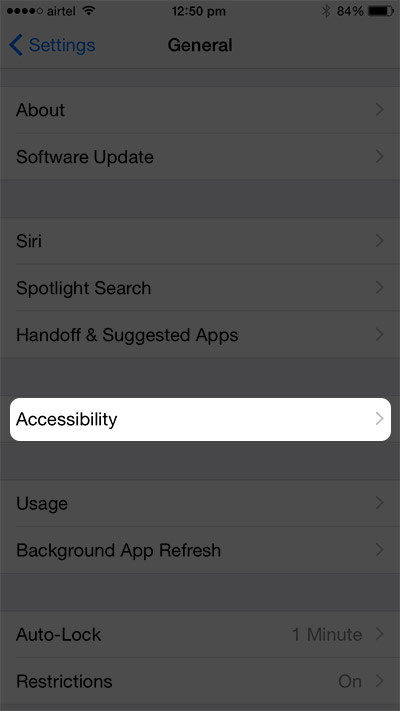This image depicts the settings screen of a cell phone, likely due to the screen layout. Notably, one line is prominently highlighted in white and stands out brightly, labeled "Accessibility" with a right-pointing arrow indicating more options. The rest of the screen is slightly dimmed and grayed out, adding emphasis to the highlighted section.

In the upper left corner, the status bar displays four out of five black dots, indicating a data signal strength, and the carrier name "Airtel" accompanied by a Wi-Fi icon. Centered at the top, the time reads 12:50 p.m. On the upper right side, icons for Bluetooth and battery life at 84% are visible.

Below this, the screen header shows "Settings" in blue font, followed by "General" in bold black font. The menu items listed beneath include "About," "Software Update," "Siri," "Spotlight Search," "Handoff and Suggested Apps," "Usage," "Background App Refresh," "Auto Lock," and "Restrictions." Each of these options is designed with a dropdown-style icon for accessing further details.